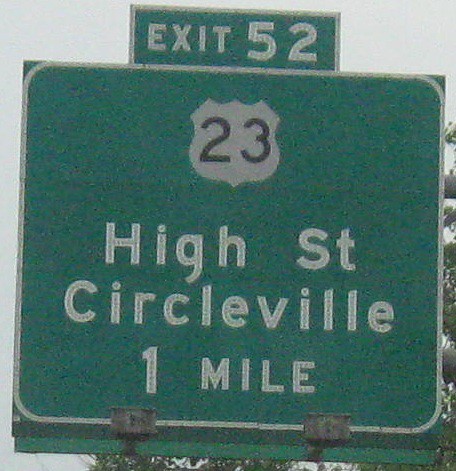A highway sign stands prominently against a backdrop of a gray, overcast sky. The upper portion of the scene features some green leaves and the partial silhouette of a tree, adding a touch of nature to the otherwise utilitarian setting. The sign itself is square and green, framed by a white border with rounded corners. Centered within the sign is a white shield emblazoned with the black number "23." At the top of the sign, above the shield, is a horizontal rectangle reading "EXIT 52" in clear, white lettering. Below the shield, the sign displays the words "High Street" followed by "Circleville" and finally "1 MILE" in descending order. The sign is mounted on two dirty gray brackets at the bottom, which secure it to a sturdy post below.